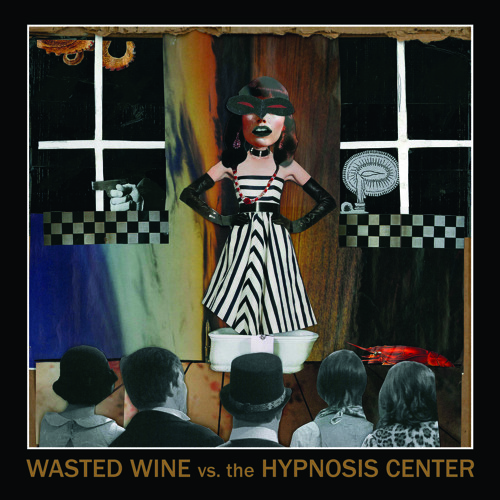This detailed Art Nouveau-inspired illustration or poster-like image is rich with dramatic and abstract elements. It features a central figure, a woman in a striking black and white striped dress without sleeves, accentuated by long black gloves that reach past her elbows. She wears a masquerade mask, which is black with red slits, obscuring her eyes, and her black hair cascades down elegantly. The woman stands on a stage, her hands confidently on her hips, with a silver bathtub or bucket behind her, further adding to the surreal nature of the scene.

The stage is set against a backdrop of a wooden wall with checkerboard patterns flanking her. This wall includes two windows: one reveals a sideways-blowing candle flame, suggesting a gust of wind, while the other depicts a disembodied hand holding a gun. This eerie tableau is observed by an audience of five people, whose backs are to the viewer, rendered in black and white. Notably, the first person on the left, a woman, wears a hat, followed by a man next to her, another man with a hat, and two additional women.

The image itself is framed within a black square border, with a thin white outline inside it. At the bottom of the black border, in gold all-capital letters, is the text "WASTED WINE," followed by "vs" in smaller lowercase letters, and then "THE HYPNOSIS CENTER" in all caps, suggesting either a title or a promotional line. Despite the overall color of the image, the audience remains in stark black and white, contrasting the vivid blue, yellow, and red hues visible in the staging elements and costumes.